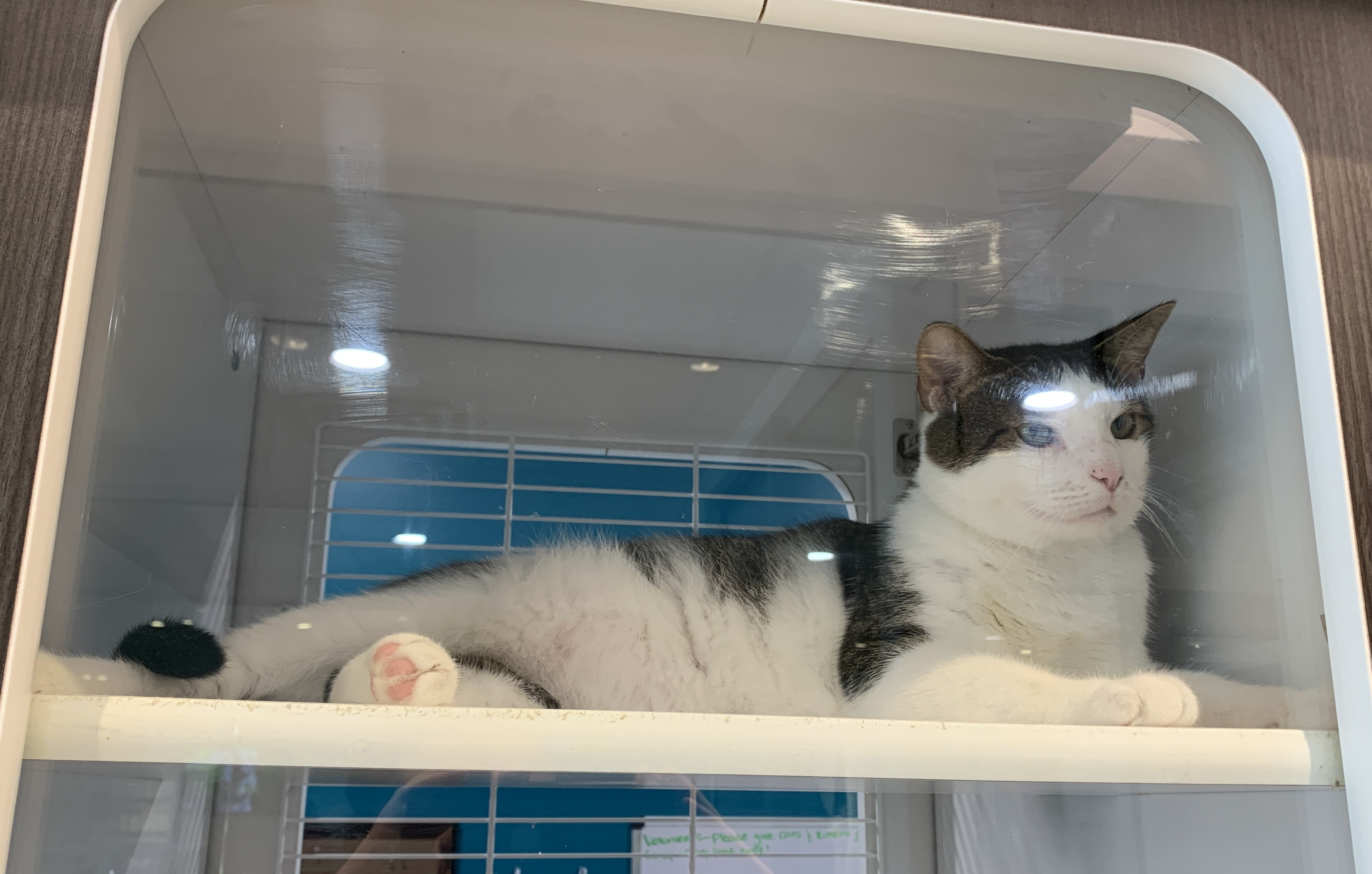The landscape-oriented color photograph depicts a detailed view of a two-level indoor enclosure, likely in a pet clinic or adoption center. The focus is on a black-and-white cat lying comfortably on the upper level of the white rectangular box. The cat's white fur adorns most of its body, contrasted with black fur on its back and a black tail. It has striking blue eyes that gaze intently towards the right side of the image. The enclosure has a glass front window, providing a clear view of the feline. At the back of the box is a clear window framed in white, and the background features a blue wall. The enclosure includes another section beneath the upper shelf, partially visible at the bottom of the image, indicating it might be part of a larger habitat possibly used for caretaker access. The cat reclines with its front paws stretched out, appearing relaxed and at ease in its contained environment.